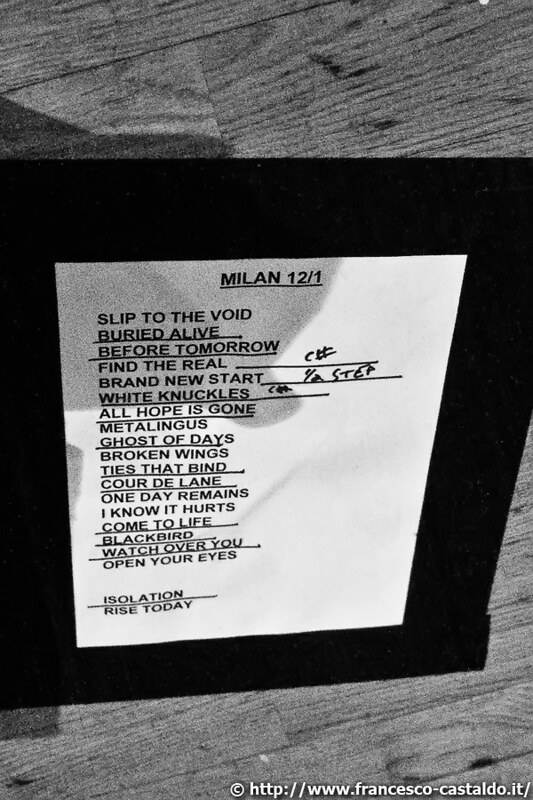This black-and-white image features a white rectangular sheet of paper, centrally placed against a black poster background, which itself is set against a wooden surface, possibly a floor or wall. The sheet, resembling a standard 9.5 by 11-inch paper, appears larger due to a prominent black border. It lists the setlist for a band, with all songs in all caps and left-justified in black lettering. At the top, it reads "MILAN 12/1," underlined. Below, the songs are listed in order: "SLIPPED TO THE VOID," "BURIED ALIVE," "BEFORE TOMORROW," "FIND THE REAL" (accompanied by handwritten "C#" notation), "BRAND NEW START," "WHITE KNUCKLES," "ALL HOPE IS GONE," "METALINGUS," "GHOST OF DAYS," "BROKEN WINGS," "TIES THAT BIND," "COEUR D'ALENE," "ONE DAY REMAINS," "I KNOW IT HURTS," "COME TO LIFE," "BLACKBIRD," "WATCH OVER YOU," "OPEN YOUR EYES," followed by a space, and then "ISOLATION," underlined, and "RISE TODAY," also underlined, indicating a possible encore. Additional handwritten notes include "HALF STEP." Shadows, possibly from a person, appear on the left of the image. In the bottom right corner, there's a small white text with a copyright symbol and the web address "http://www.francesco-castaldo.it."